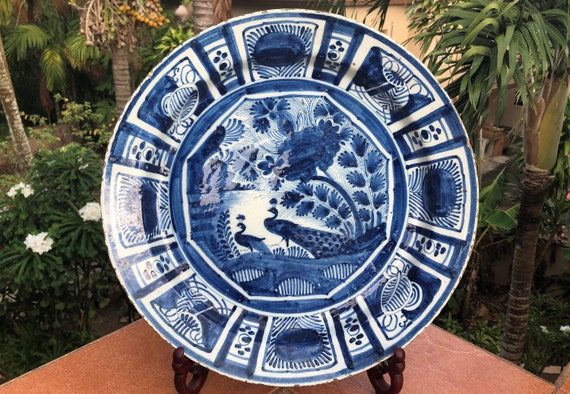This decorative blue and white china plate, intricately designed and on display, rests on a dark wooden stand on a brown table. Set outdoors amidst a backdrop of blossoming bushes and palm trees, the plate captures a picturesque scene within its craftsmanship. The inner border features two majestic peacocks with long tails, walking amidst blue trees and floral elements, conveying a garden-like ambiance. The peacocks appear to be walking across a bridge, framed by the foliage. The outer border of the plate is adorned with an array of etched shapes, including leaves and flowers, presented in various textures and sections. The detailed artistry of peacocks, trees, and floral motifs extends throughout the plate, creating a harmonious and visually stunning piece on an elegantly simple wooden stand.